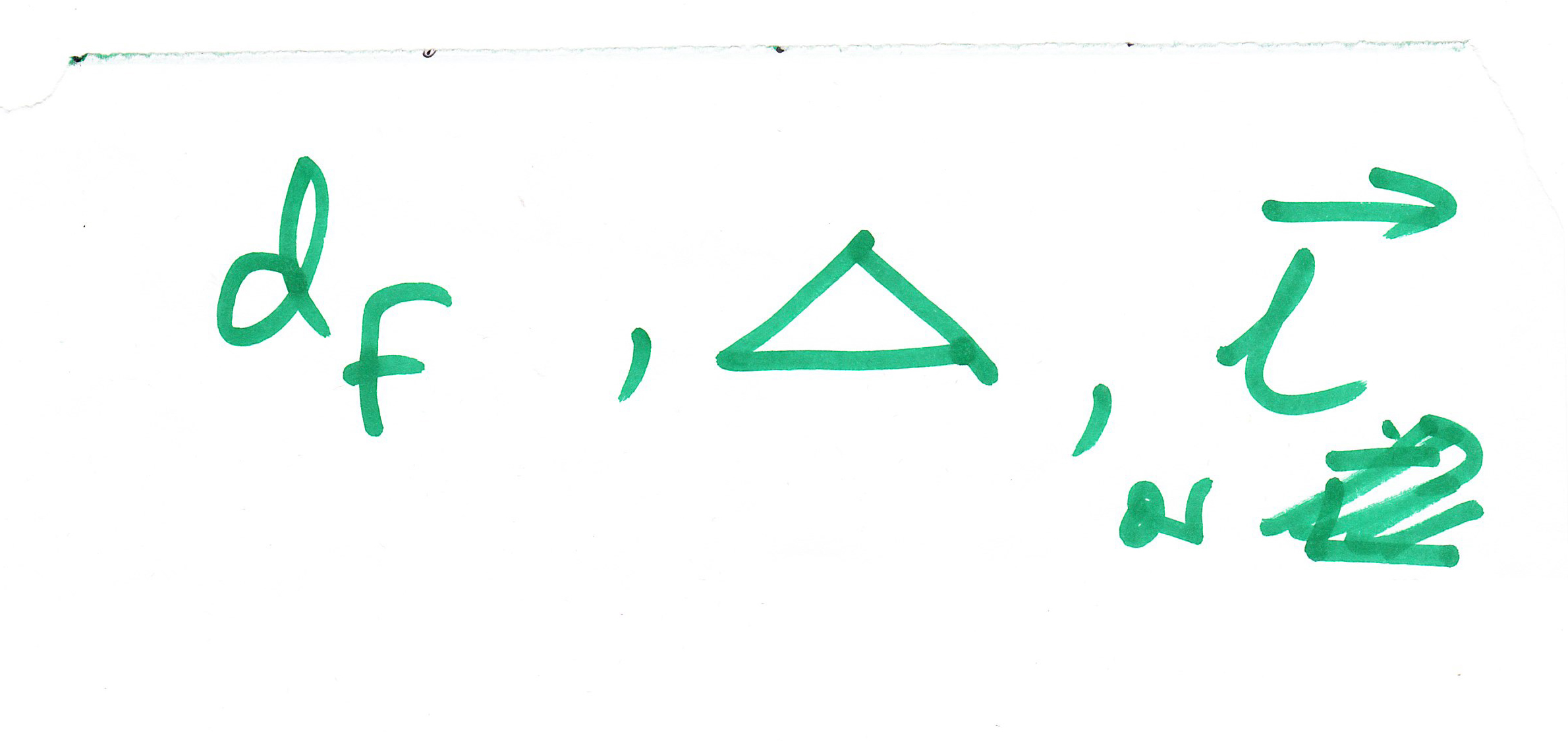The image shows a scanned piece of paper with various symbols written in dark green ink, likely from an alcohol-based marker, as evidenced by the varying intensity of the ink. At the top of the page is a horizontal ink stain, possibly the edge of the paper or another ink blemish. The symbols are arranged from left to right and include: the letter "D" followed by a capital "F" positioned at the bottom right, suggesting a possible math notation of "D raised to the power F." This is followed by a comma, a crudely drawn triangle, and a second comma. Next, there is a right-pointing arrow with a cursive "L" beneath it. Below the cursive "L," two additional symbols appear to be crossed off, making them difficult to interpret.